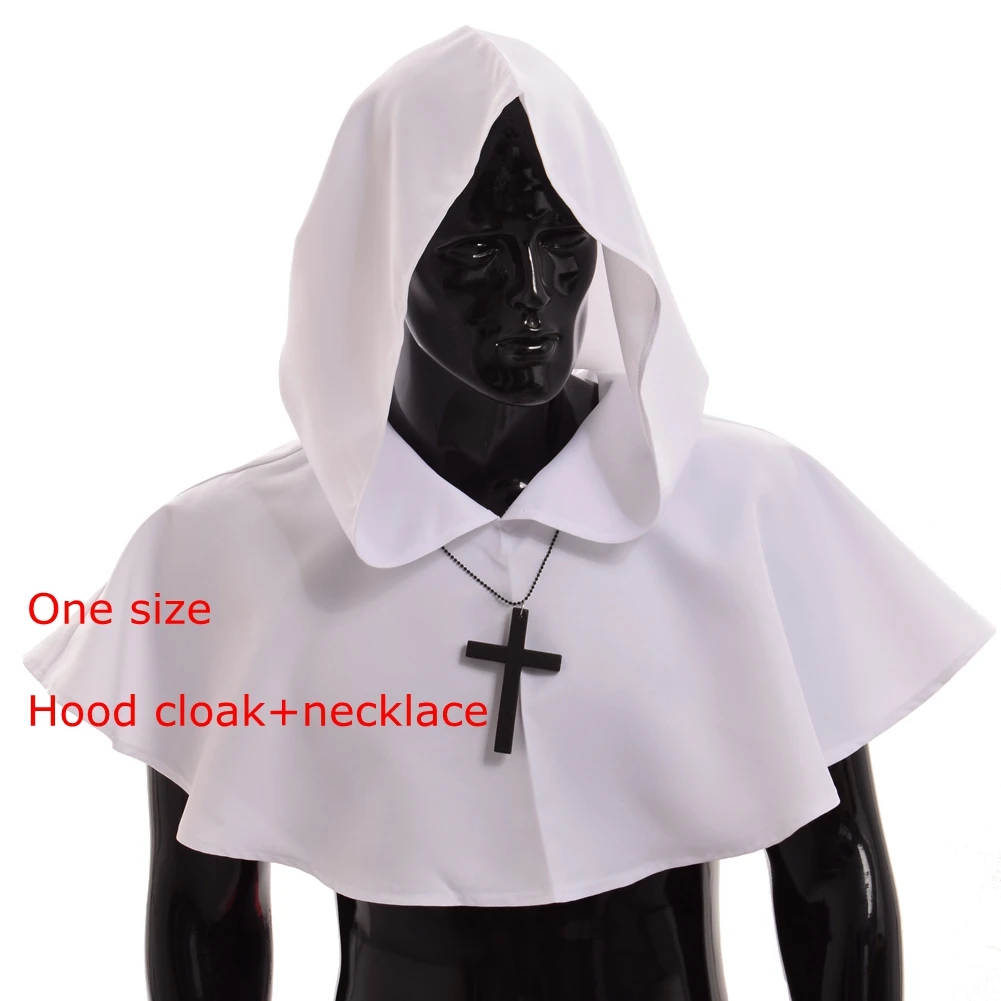This indoor photographic image showcases a black mannequin adorned in a religious-inspired outfit. The focal point of the ensemble is a white hooded cloak that extends just past the chest, revealing the midriff. The mannequin is also adorned with a striking black cross necklace, featuring a bead chain, with the cross itself measuring approximately five to six inches long and four inches wide. The mannequin's head is slightly tilted downward and away from the camera, emphasizing the cloak and the necklace. Notably, red text on the left side of the image reads "one size, hood, cloak, and necklace," indicating these components are likely part of a singular costume set. The overall setting appears minimalist with a plain white background that accentuates the contrast between the black mannequin and the white outfit. The precise and detailed design suggests the attire could be suitable for a religious role, such as a priest or nun, but it might also be aimed at costume applications, like for Halloween.